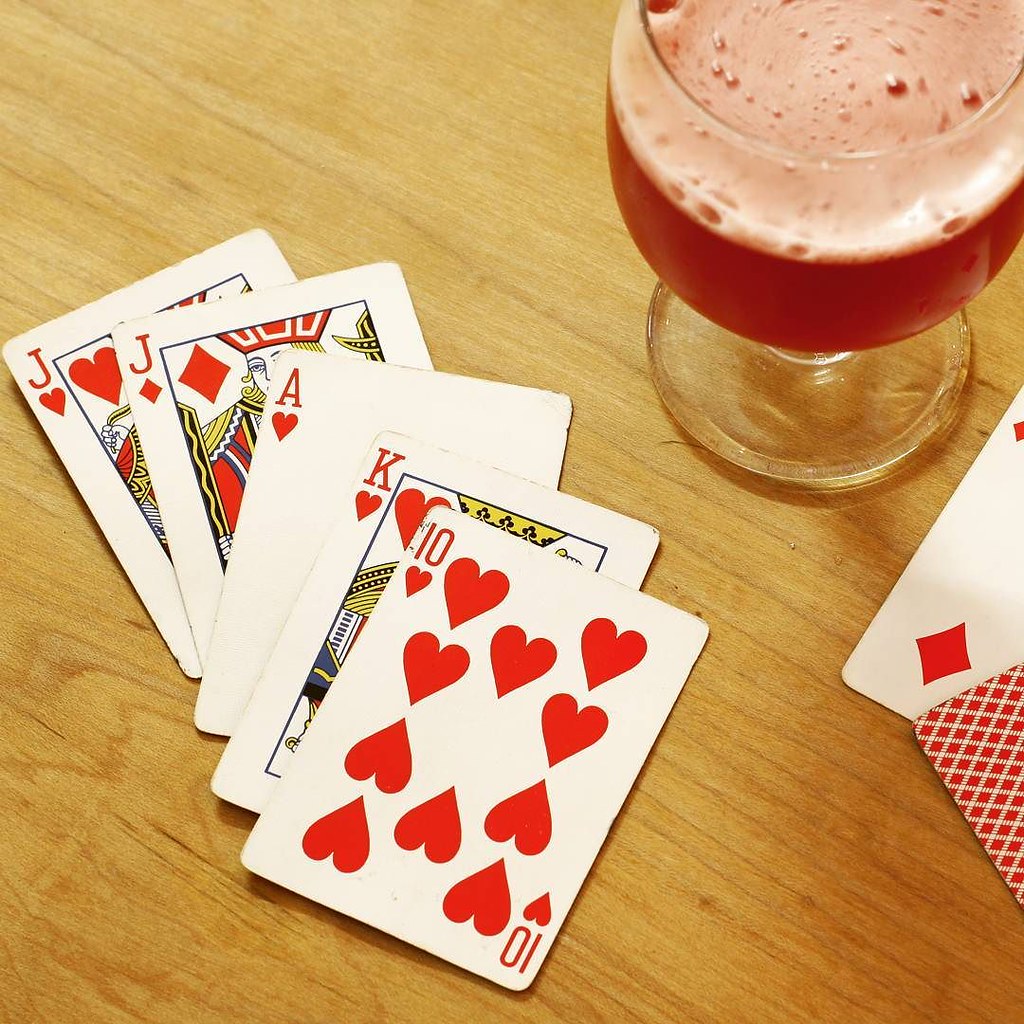This overhead shot captures an intimate scene, likely set in the cozy kitchen of someone's home. The focus is on a portion of a light honey oak kitchen table, with its natural grain patterns and occasional dark indentations akin to scratches subtly highlighted by the play of light and shadows.

The centerpiece of the image is a wine glass with an elegantly slender stem and a broad, rounded bowl. The glass holds a frothy reddish-pink beverage, though the exact hue is somewhat ambiguous due to the lighting—there are hints of a lighter, almost swirled white froth sitting atop the drink.

Scattered around the glass are playing cards, hinting at a paused or leisurely game. Visible cards include a Jack of Hearts, Jack of Diamonds, Ace of Hearts, King of Hearts, and Ten of Hearts, stacked partially over one another. To the right, an additional card—and another with its red back facing upwards—adds to the scene's casual, lived-in charm, suggesting an engaging evening activity.